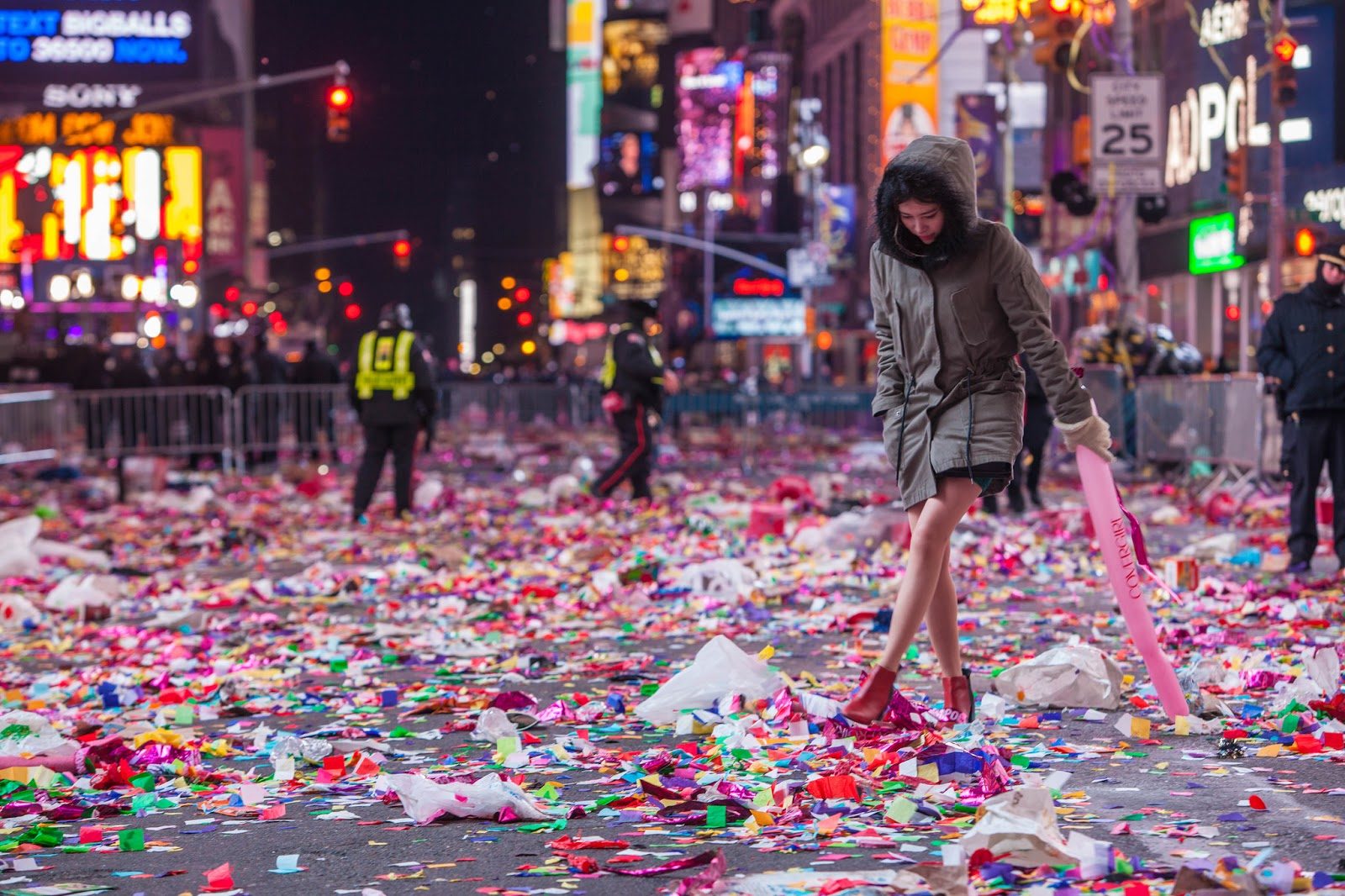This nighttime photo, likely set in Times Square, New York City, captures the aftermath of a festive celebration. The focal point is a young woman wearing a gray winter coat with a fur-lined hood, red shoes, and a pair of gloves, but oddly, no leggings. She seems to be interacting with the confetti-strewn ground, possibly kicking or inspecting it. The confetti, scattered across the entire fenced-off area, is an array of vibrant colors, including pinks, blues, greens, and whites, alongside some discarded party items. Nearby, various police officers and security personnel in yellow vests patrol the area. Noteworthy in the background are the high-rises adorned with city lights, multiple signs including a speed limit sign for 25, and prominent advertisements such as a Sony billboard. A red traffic light is also visible, reinforcing the urban setting of this lively yet now tranquil scene.